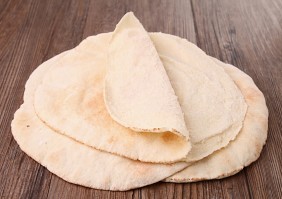This detailed indoor color photograph showcases a stack of flat bread, possibly pita or tortillas, centered prominently on a dark brown wooden table. The stack comprises four to six pieces, most of which are slightly askew, with the bottom two off-center. The top piece is folded in half with the fold pointing left. The flatbread is light in color with subtle textural variations, giving it a fluffy and slightly puffy appearance. The edges are not perfectly circular, adding a rustic charm. The wood grain of the table is clearly visible, providing a contrasting backdrop to the light-colored bread. The lighting is soft, highlighting the texture and thickness of the flatbread without casting harsh shadows, making the bread appear particularly appetizing. There are no additional objects or text within the frame, allowing the viewer’s focus to rest solely on the appealing stack of bread.